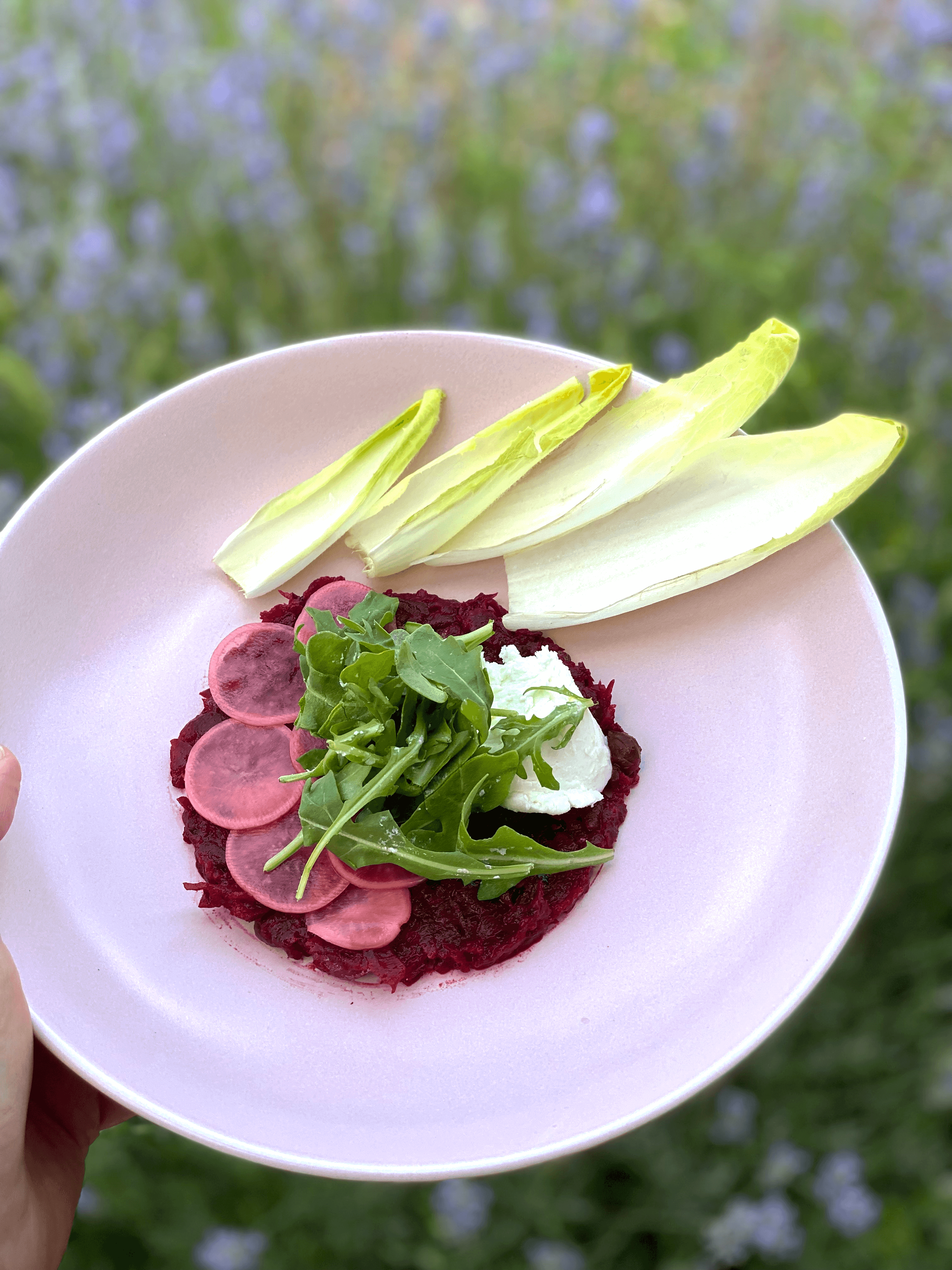In the foreground, a hand is partially visible, holding up a white plate with a tantalizing array of culinary elements. The central focus of the dish is a dollop of vibrant red paste. To the left, delicate slices of a light pink item, likely salmon or a similar seafood, are neatly arranged. Occupying the middle section, an abundance of deep green leaves, possibly radicchio, adds a burst of color and texture. On the right side of the plate, a generous spoonful of creamy white substance, likely a cheese or yogurt-based element, balances the composition. Draped over the entire assembly, slender, pointed leaves resembling endive or another type of lettuce lend an artistic and structural flair to the presentation. The blurred background hints at an outdoor setting, with indistinct shapes suggesting sky and trees, further emphasizing the fresh and vibrant theme of the dish.